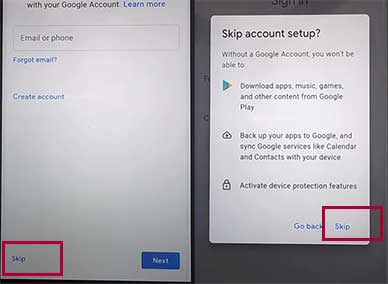This is a partially-captured photo of a Google Account setup tab on a desktop screen. At the top left corner, it displays the title "With your Google Account" and a "Learn more" link highlighted in blue. Below this title, there is a text box labeled "Email or phone," and to the left underneath this box, there is a "Forgot email?" link in blue. Centered on the page, there is also a "Create account" link. At the bottom of the page, there are two buttons: a red-edited box over the "Skip" button on the left and a blue "Next" button on the right. Additionally, on the right side of the screen, there's a pop-up titled "Skip account setup," explaining that without a Google account, users won't be able to download apps or backup their apps. The pop-up also has two options: "Go back" or "Skip." The "Skip" option is highlighted with a red-edited box. It appears that the person took a screenshot to create a tutorial, emphasizing the "Skip" options with added red boxes to guide someone on how to bypass the account setup process.